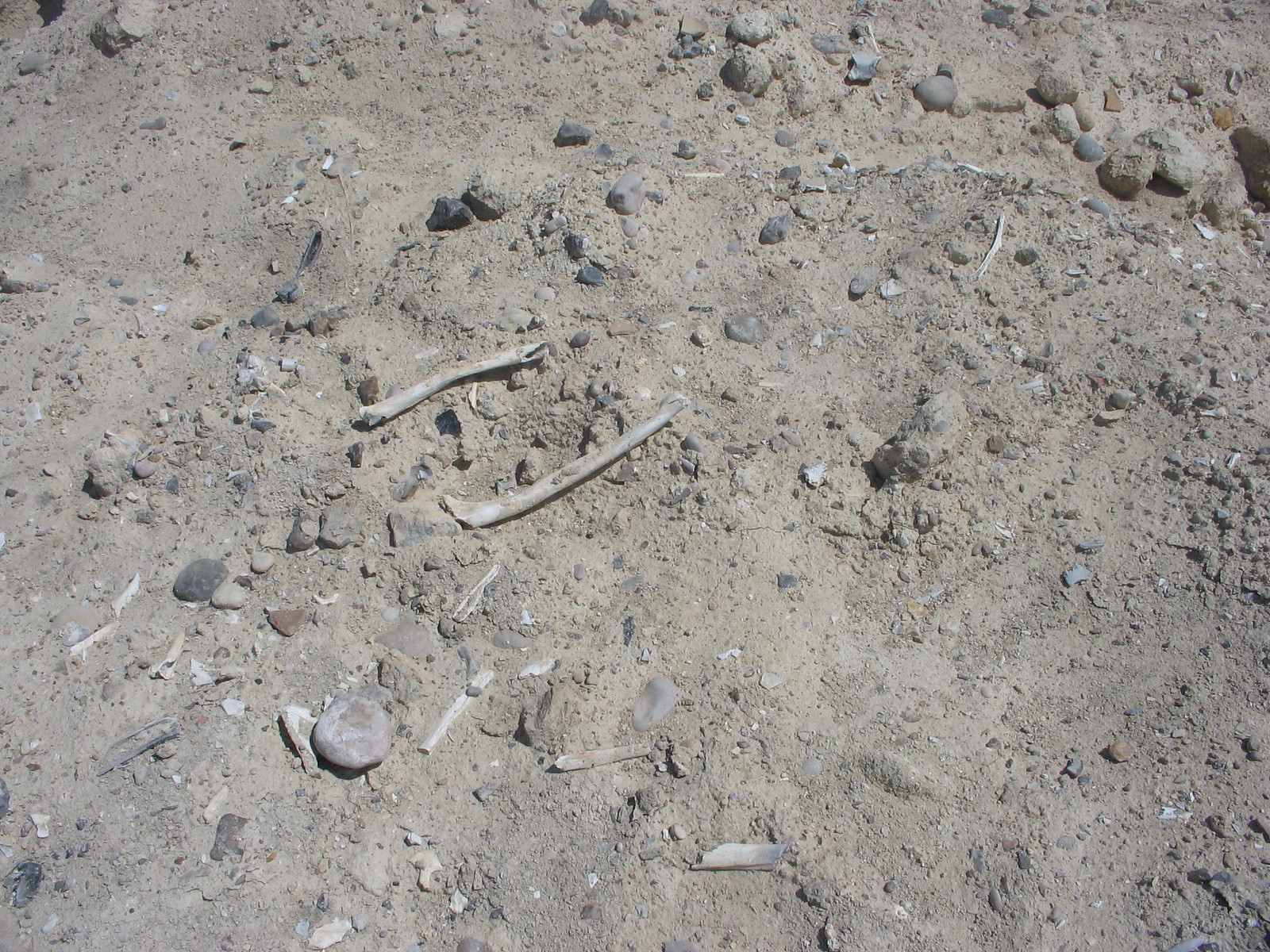The image depicts a barren, gravelly landscape with uneven ground, characterized by a mix of gray and brown hues. Scattered rocks of various sizes, from small, jagged chunks to larger, rounded stones, are strewn across the scene. Amidst this rough terrain, a pair of prominent bones, covered in dust and appearing somewhat gray, lie parallel to each other near the center. The upper bone displays a visible fracture at one end, casting a black shadow within. Surrounding these bones, smaller bone fragments and slivers, also dusty and in shades of gray, yellow, and white, are dispersed haphazardly across the ground. The area appears desolate and dry, with certain sections revealing slight furrows that hint at past water flow, accentuated by clusters of round rocks. The overall setting resembles a desolate outdoor scene, possibly near a beach, due to the sandy and gravelly texture of the terrain.